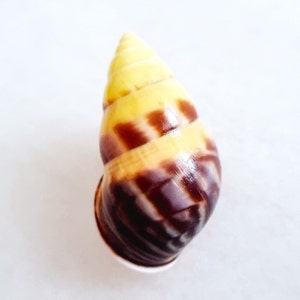The image depicts a close-up of a snail shell positioned against a white background. The shell features a distinct spiral tip and showcases a color gradient that transitions from a brown base to a yellow top, marked by a single brown stripe in the middle. The shell, which appears to be about the size of two quarters, is gleaming brightly, particularly on the upper right-hand side where the light reflects off its surface. The base of the shell is facing downward, making the interior of the shell invisible. The white tabletop accentuates the clear, vibrant details of the shiny shell, which stands out prominently in the picture.